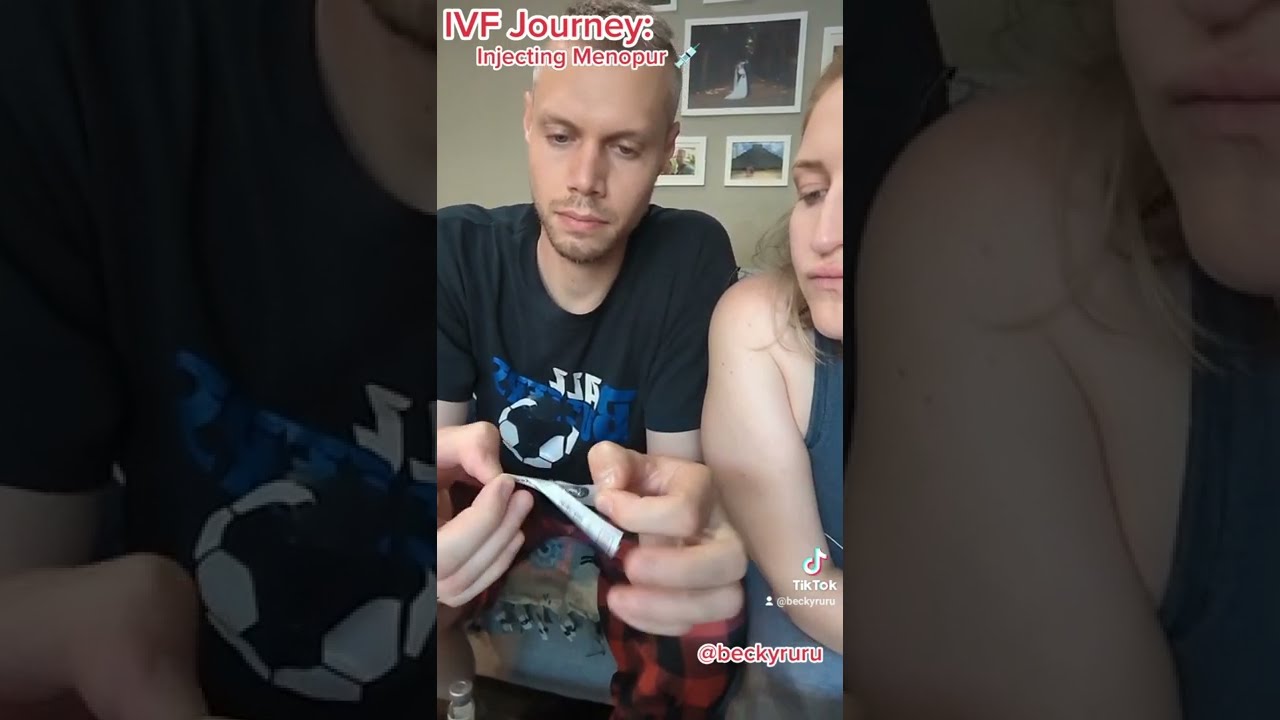In the center of this wide rectangular image, there is a tall vertical photograph showing a man and a woman intently looking down at a piece of paper. The man, on the left side, has light brown hair and a very narrow beard and mustache. He is wearing a black shirt that features a soccer ball emblem and red checkered pants. The piece of paper he is holding is grasped between his thumb and index finger on both hands. The woman sits to his right, also focusing on the paper. She is wearing a blue tank top and has blonde hair. Above the man, in red letters with a white outline, the text reads "IVF Journey: Injected Menopur." In the bottom right corner, the TikTok emblem is displayed along with the handle "@BeckyRURU." Behind them, a gray-colored wall is adorned with several pictures in white frames. The central picture, visible directly between their heads, appears to depict a person wearing a wedding dress. The left and right sides of the wider rectangular image are tinted close-up zooms of the central photograph, emphasizing the details of the scene.